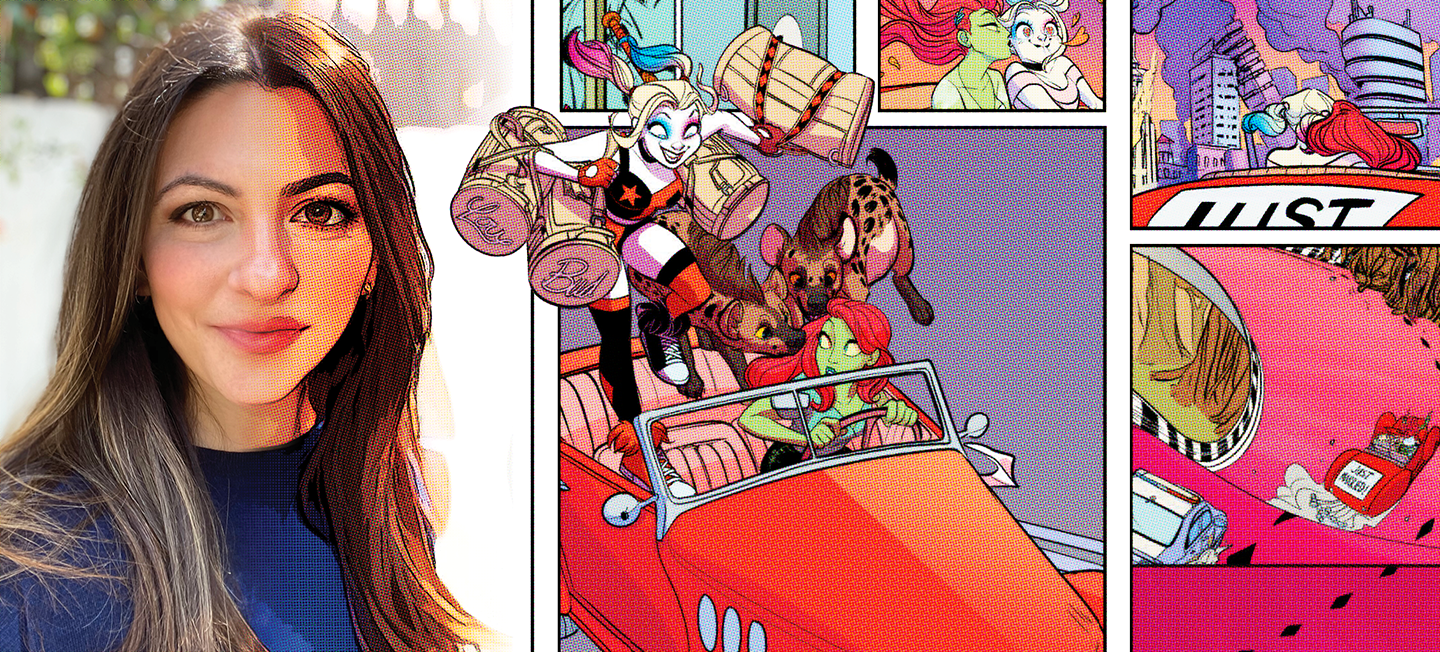The image is divided into three distinct panels, blending realistic and comic book styles. The leftmost panel features a woman with long brown hair, brown eyes, and rose-colored lips. Her appearance transitions from normal on the left side to a cartoon-like representation on the right, set against a white background. The central panel is a lively comic scene: a woman with red hair and green skin drives a red car, accompanied by another woman carrying four bags labeled "love" and "bud." Two hyenas are seen trying to jump into the car, which has a "just married" sign on it. In the top-right part of the central panel, there is a close-up of this sign. The rightmost panel continues the comic narrative with smaller images, including a scene of two women kissing, one in green with red hair and the other in a pink top, with a burning building and a car driving away in the background. Overall, the image juxtaposes realistic and cartoon elements, creating a compelling, multi-layered visual story.